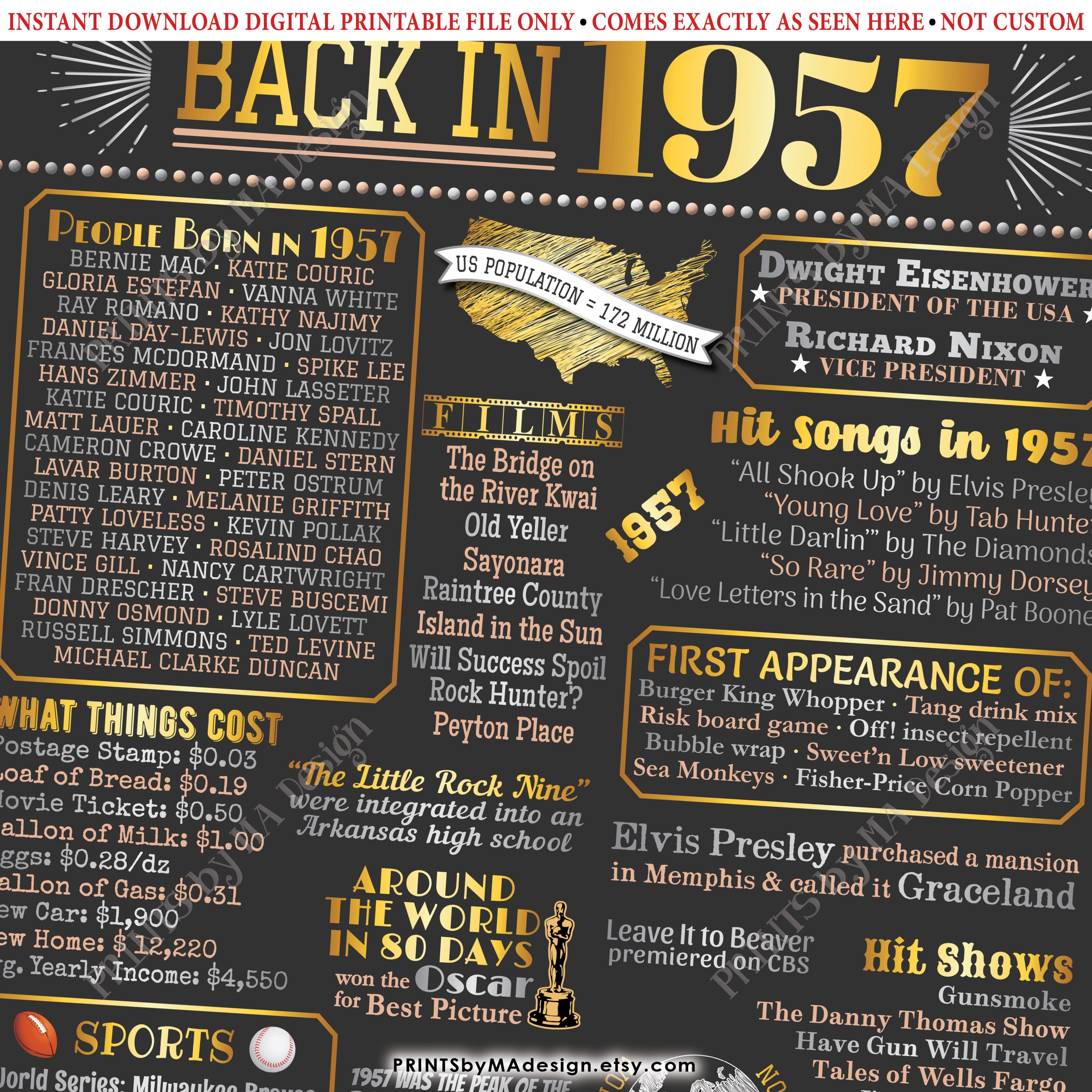This image is an instant download digital printable file, presented exactly as shown without customization, set against a dark gray background with various striking and bold letterings. At the top in gold, the header states "Back in 1957" alongside a golden illustration of the US map, highlighting the population at that time as 172 million. The image is rich with historical details, encapsulating notable events, entertainment, and cultural facts from the year.

Key sections include:
- **People Born in 1957:** Lists of famous individuals born that year.
- **What Things Cost in 1957:** Prices of various commodities and groceries.
- **Sports:** Highlights from the year's sports events, though partially cut off at the bottom.
- **Films:** Movies released in 1957, including the Oscar-winning "Around the World in 80 Days."
- **Television and Music:** Premieres of shows like "Leave It to Beaver" and hits of the time, with specific mentions of Dwight Eisenhower as President and Richard Nixon as Vice President.
- **Cultural Milestones:** Includes events like the integration of the Little Rock Nine into an Arkansas high school, Elvis Presley's purchase of Graceland, and the debut of products such as the Risk board game, Bubble Wrap, Sea Monkeys, and the Burger King Whopper.

The design is meant to captivate and inform, giving a comprehensive snapshot of the year 1957 through a visually engaging and information-rich format.